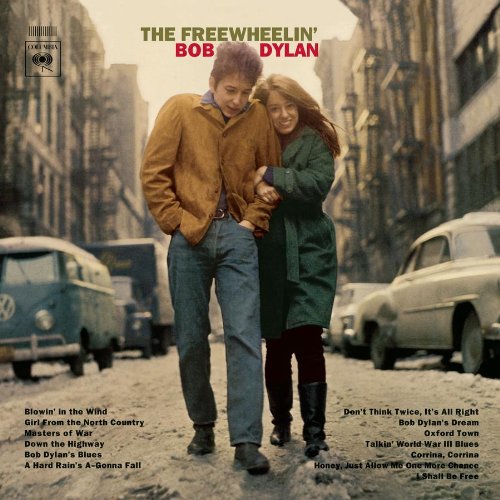The image is the back cover of the album titled "The Freewheelin' Bob Dylan." The title "The Freewheelin'" is written in green, while "Bob Dylan" is in red, both centered towards the top. Below the title, there's a photograph of Bob Dylan and his girlfriend walking down the center of a street in what appears to be New York City, likely in the Union Square or Greenwich Village neighborhood. The street is flanked by city buildings and various vehicles, including a Volkswagen van and a big blue truck on the left side, seemingly moving towards the viewer, and other parked cars on the right side, moving away.

In the photograph, Dylan is wearing a brownish coat, blue jeans, and black shoes, with his hands in his pockets and his hair tousled. His girlfriend, holding on to his left arm, has shoulder-length hair and is wearing a green coat that resembles a dress, black pants, and black boots up to her shins. The ground is covered with a bit of snow, adding to the scene's wintry feel.

Towards the bottom of the cover, the song listings for the album are displayed, with side A on the left and side B on the right. Side A includes "Blowin' in the Wind," "Girl from the North Country," "Masters of War," "Down the Highway," "Bob Dylan's Blues," and "A Hard Rain's A-Gonna Fall," while side B features "Don't Think Twice, It's All Right," "Bob Dylan's Dream," "Oxford Town," "Talkin' World War III Blues," "Corrina, Corrina," "Honey, Just Allow Me One More Chance," and "I Shall Be Free."